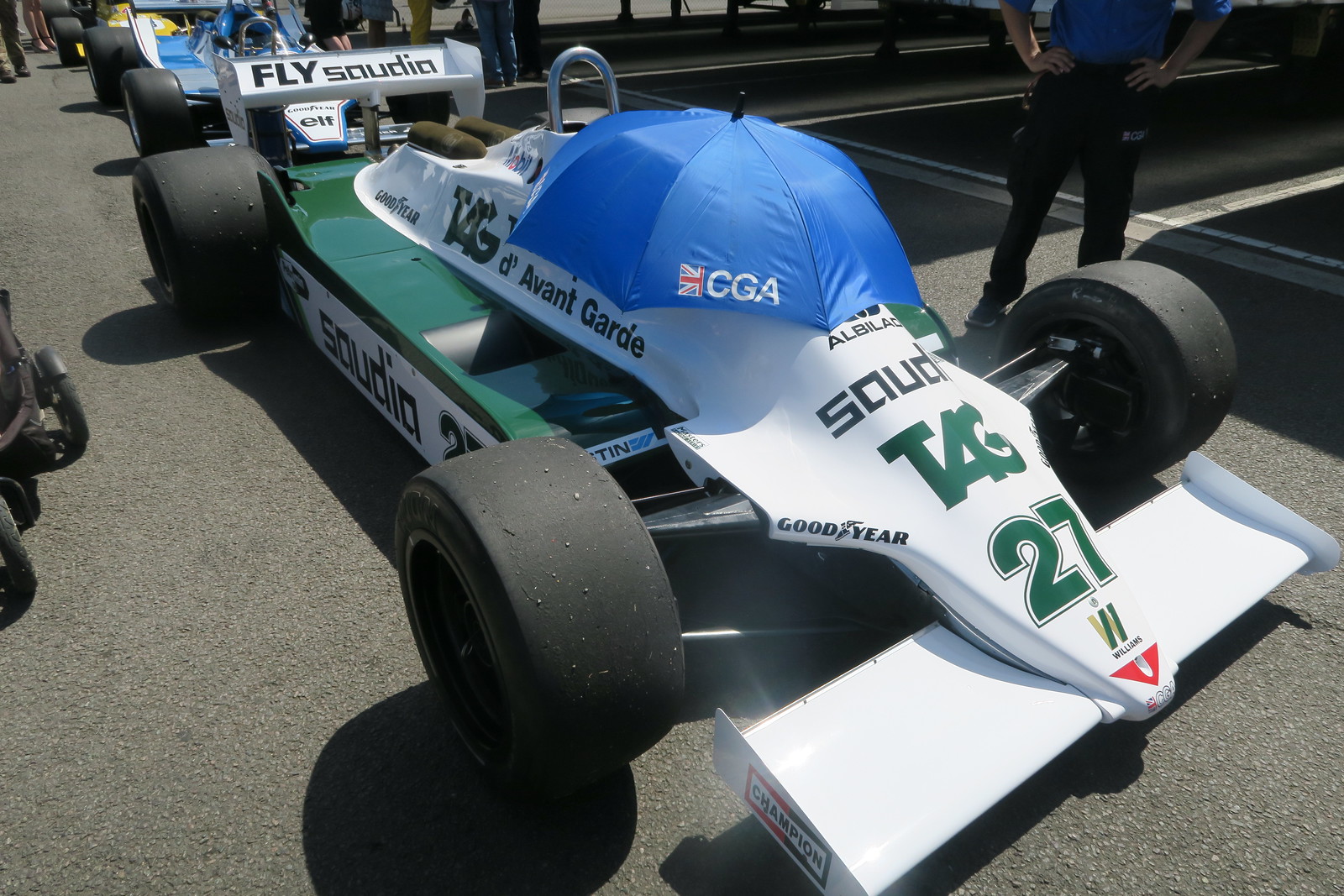The image depicts an IndyCar, or possibly a similar Formula racing car, positioned on black asphalt, likely in the pit area before a race. The car itself is predominantly green with white accents near the cockpit area. All four black, round wheels are visible, although the right wheel is partially obscured by the vehicle's body. A notable feature is a blue umbrella with 'CGA' in small white text and part of a British flag, positioned atop the cockpit. Additionally, the car is adorned with various sponsor logos, including 'Saud' in black text at the front, 'Tag' in green text just below that, followed by the number '27' also in green. 

To the top right of the image, a man is visible from the shoulders down, dressed in a blue shirt and black pants, with his hands on his hips. In the background on the top left, another similar IndyCar, mainly blue with white trim, is visible. The scene is well-lit, highlighting the asphalt around the vehicles. The green car casts a shadow, emphasizing the contrast between the vibrant colors of the car and the dark tarmac.